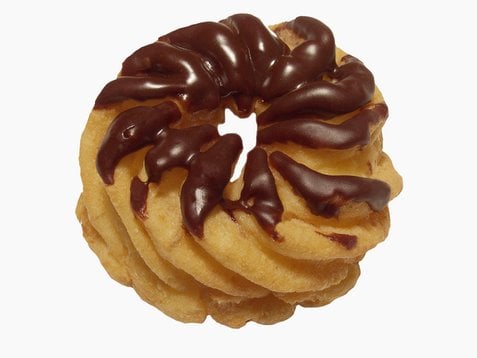This image features a single prominent object centered on an eggshell white background, typical of what might be seen in an online shop or bakery website. The object is a large, circular donut made from a dough reminiscent of old-fashioned donuts but designed with unique spiral swirls and small cavities between each swirl, giving it a more intricate texture. The donut's hole is quite small, and its light brown surface is adorned with a thin layer of glossy, dark brown chocolate icing, which is thicker at the top and thinner toward the bottom. The icing's sheen suggests it has been freshly applied, adding to its appetizing appearance. The scene is minimalist, with no other objects or text in the frame, focusing entirely on the detailed presentation of the donut.